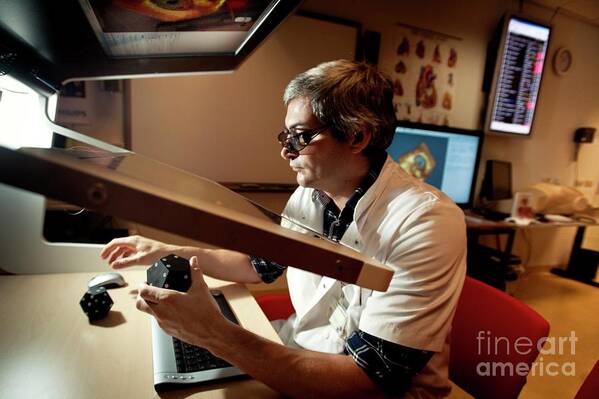The photograph is taken indoors, possibly in a laboratory setting. It shows a room with tables in the background. On the right-hand side, there's a large computer monitor on one of the tables. On the left-hand side, at another table, a middle-aged man is seated, appearing to be a scientist. He is dressed in a white lab coat over a rolled-up, long-sleeve shirt and is wearing eyewear. In his hands, he is holding a large black dodecahedron, with another similar object on the desk in front of him, near a keyboard. There is a glass panel lifted above him. The bottom right-hand side of the image features white lettering that reads "Find Art America." The overall scene suggests a scientific environment where the man is possibly examining or reviewing the dodecahedron-like objects.